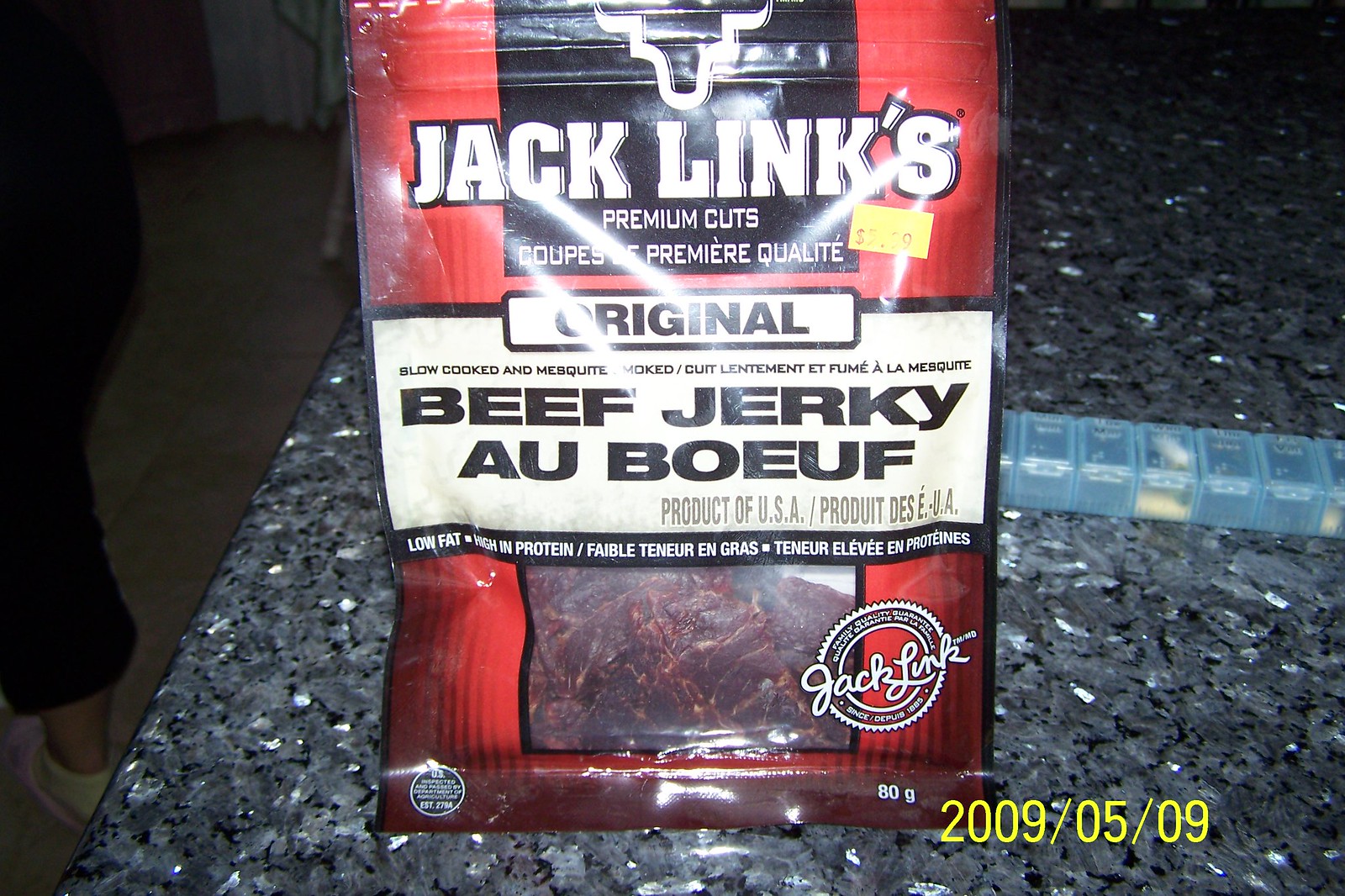The image showcases a package of Jack Link's Original Beef Jerky prominently displayed on a gray, black-flecked countertop, likely in a kitchen setting. The packaging is predominantly red with black and yellow accents, featuring a clear section that reveals the brown beef jerky inside. The top of the package bears the Jack Link's logo in white text on a black background, accompanied by a bull head icon. Below the logo, a white bar with black text reads "Original Beef Jerky." Additional text indicates "Premium Cuts, All Beef, Product of USA," with some French phrases suggesting the packaging might be intended for sale in France. A pill divider sits behind the jerky, and a date stamp in yellow text, reading "2009/05/09," is visible in the bottom right corner of the image.